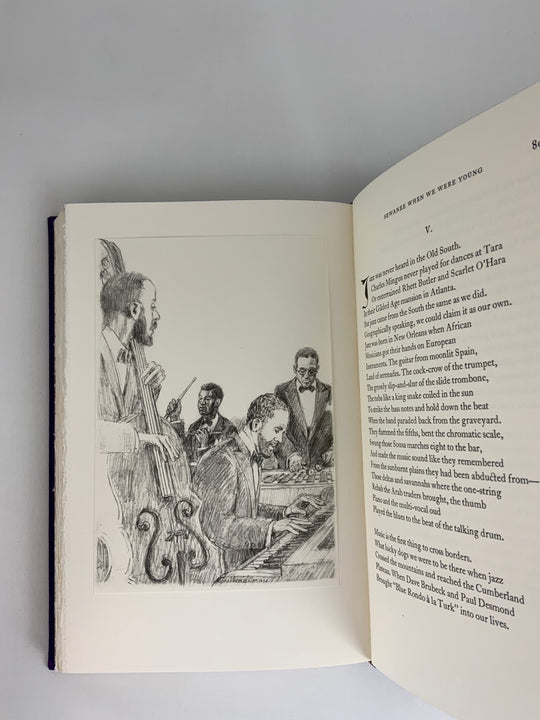The photograph captures an open book resting on a light grey surface that almost appears white. The book features an illustration on the left page and text on the right. The left page showcases a detailed, hand-drawn black and white illustration of a vintage jazz band. The band comprises a bassist on the left, a pianist in the middle, a drummer in the background holding a drumstick, and another standing musician on the right. All the musicians are dressed in formal attire, wearing suits or tuxedos with bow ties. The right page contains text written in black, including a header at the top and a page number on the upper right. There's also a Roman numeral "V" or the letter "V" placed centrally at the top. The text describes the Jazzmen in Atlanta, focusing on the 1940s to 1950s era. The book itself has white pages and appears to have a black cover.